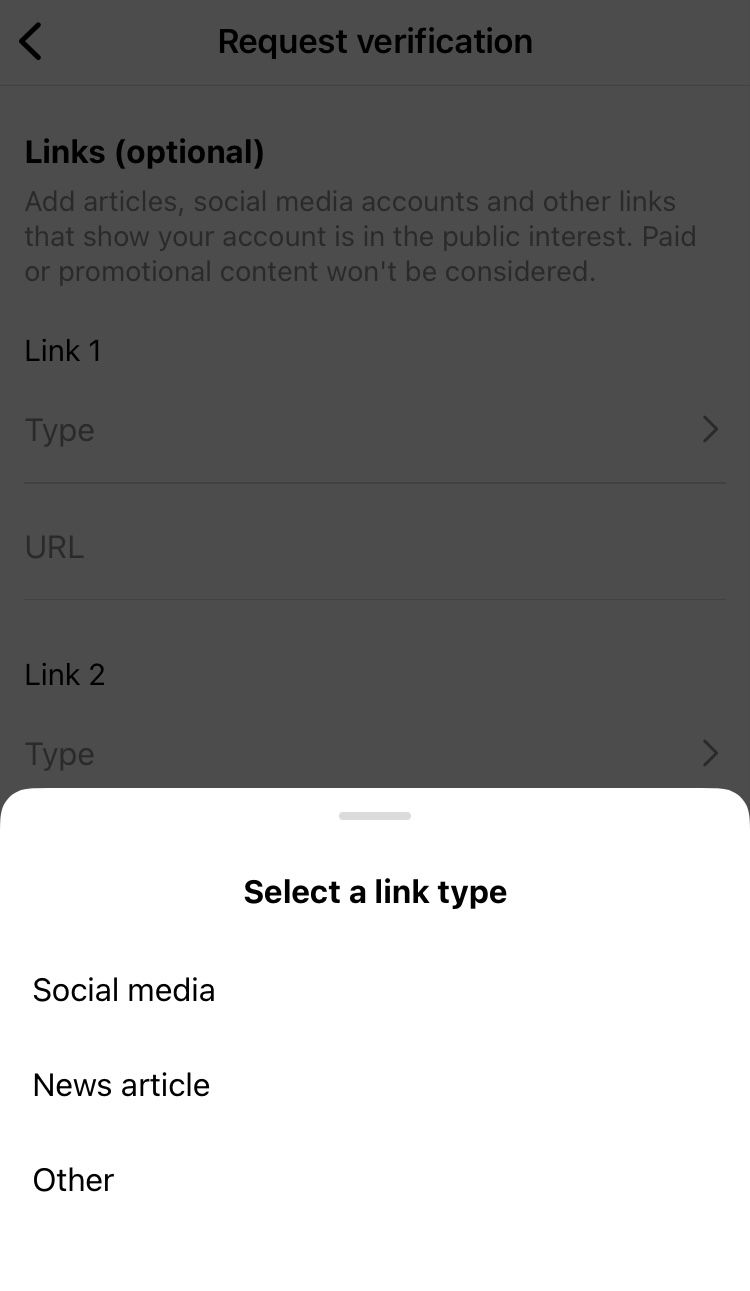This vertically oriented rectangular image features a structured layout with a mostly gray background at the top. At the uppermost center, the heading "Request Verification" is prominently displayed in bold black font, with only the first letter of "Request" capitalized.

In the upper left corner, a small left arrow is present. Below this, the text "Links (optional)" is written in bold black font, with the word "Links" capitalized and the term "optional" in lowercase enclosed in parentheses. The instructions beneath this header emphasize the need to "add articles, social media accounts, and other links that show your account is in the public interest," clarifying that "Paid or promotional content won't be considered."

Further down, the document details an entry field labeled "Link 1" in bold black font. Under this, the placeholder "type" (T-Y-P-E) appears in light gray font. To the far right, a small right-pointing arrow is visible. On the left underneath the placeholder, the acronym "U-R-L" is written in all capital letters.

Below, the format repeats with a similar entry labeled "Link 2," followed by "type" in a possibly black but not bolded or gray font. To the right is another right-pointing arrow.

A second section begins below, marked by a thin light gray horizontal line in the top center of a white background. "Select a link type" is stated in black bolded font, again with only the "S" in "Select" capitalized. The section lists "social media," "news article," and "other" in black font, each separated by a blank line.